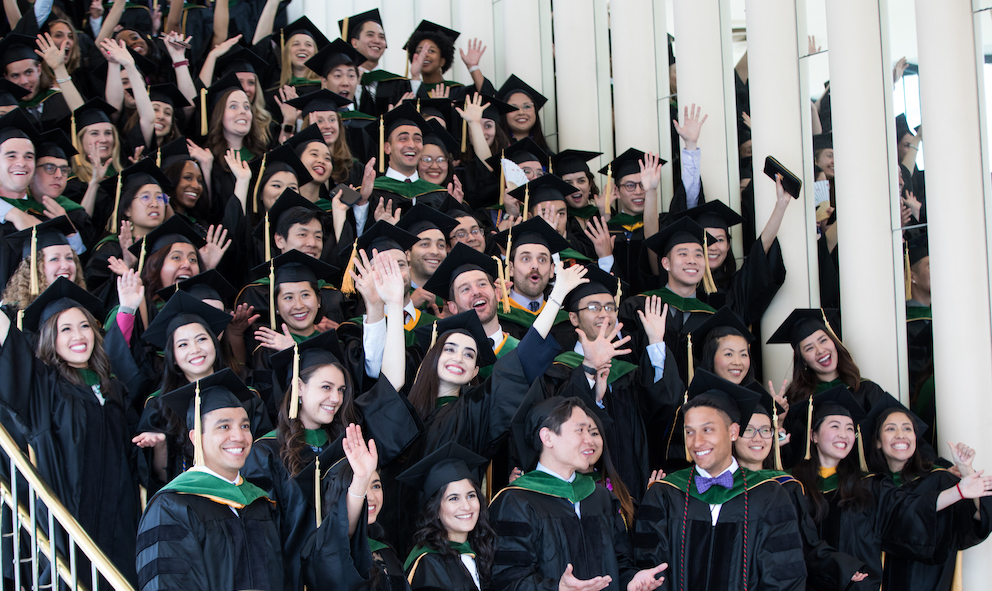In this celebratory real-life photo, over 50 joyful college graduates, possibly from a prestigious and accredited institution, are captured standing on a wide metal staircase that tilts at a 45-degree angle from the top left to the bottom right of the picture. They are all adorned in traditional black graduation gowns and caps with yellow tassels, complemented by green sashes with gold trim draping over their shoulders. The vibrant group is enthusiastically waving their hands at something off to the right, their faces glowing with happiness. The staircase has a handrail visible at the bottom left, and the side wall is lined with mirrors that reflect the excited crowd. The combination of their uniform attire, the orderly yet dynamic arrangement on the stairway, and their cheerful demeanor collectively convey the elation of this significant milestone.